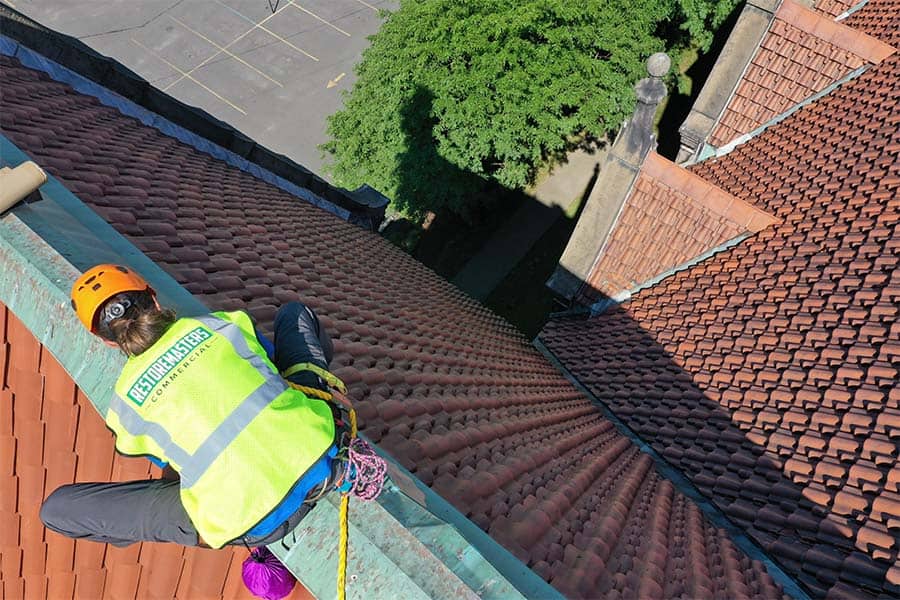This detailed aerial color photograph, likely taken by a drone, captures a female worker straddling and leaning over a steep, reddish-orange, terracotta-style roof that features the characteristic Mediterranean plates. The roof dramatically slopes to almost a 90-degree angle on the right side, while the left side has a gentler incline. The worker is identifiable by her bright yellow safety vest with reflective tape, a green rectangle with white letters reading "Restore Masters," and the word "Commercial" in black text beneath. This vest also has a gray rectangle outline surrounding the text. 

She is equipped with a safety harness with red ropes around her waist, wearing an orange safety helmet, grayish-black pants, and has her hair up in a bun. A small purple satchel hangs from her left side. Surrounding the roof are several notable elements: trees at the bottom, a parking lot in the top left corner, a line of additional trees at the top, and another orange and red roof section connecting at the 90-degree drop. Two archways are visible, with one arch featuring a small statue.